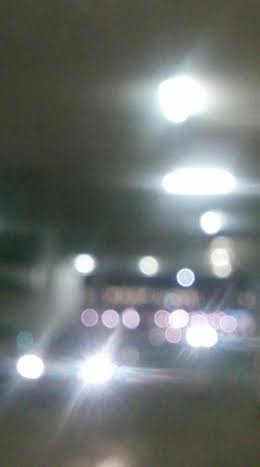The image presents a highly distorted and blurred vertical photograph that is challenging to discern clearly. Dominating the scene is the blinding glare of headlights from an approaching large diesel-like truck, suggesting a feeling of imminent collision. The truck's large, white body is vaguely visible amidst the pervasive brightness. Above, a series of large, wide ceiling lights, resembling tunnel lighting, contribute to the intense overall illumination. The background harbors a dark, blackish-green hue, blending into the dim foreground. Across the image, various rows of circular lights—ranging from light pink to pure white—are distributed unevenly, adding to the chaotic atmosphere. In the upper part, two large white lights shine prominently, evoking the intensity of stadium lights. Additional light elements include halos and rows of smaller lights mingling with the primary scene. Some lighter-colored, rectangular objects, possibly buildings or other structures, are faintly visible between the rows of lights in the center. Overall, the mixture of bright headlights, ceiling lights, and abstract shapes creates a heavily distorted, almost surreal visual effect, making it difficult to distinguish finer details.